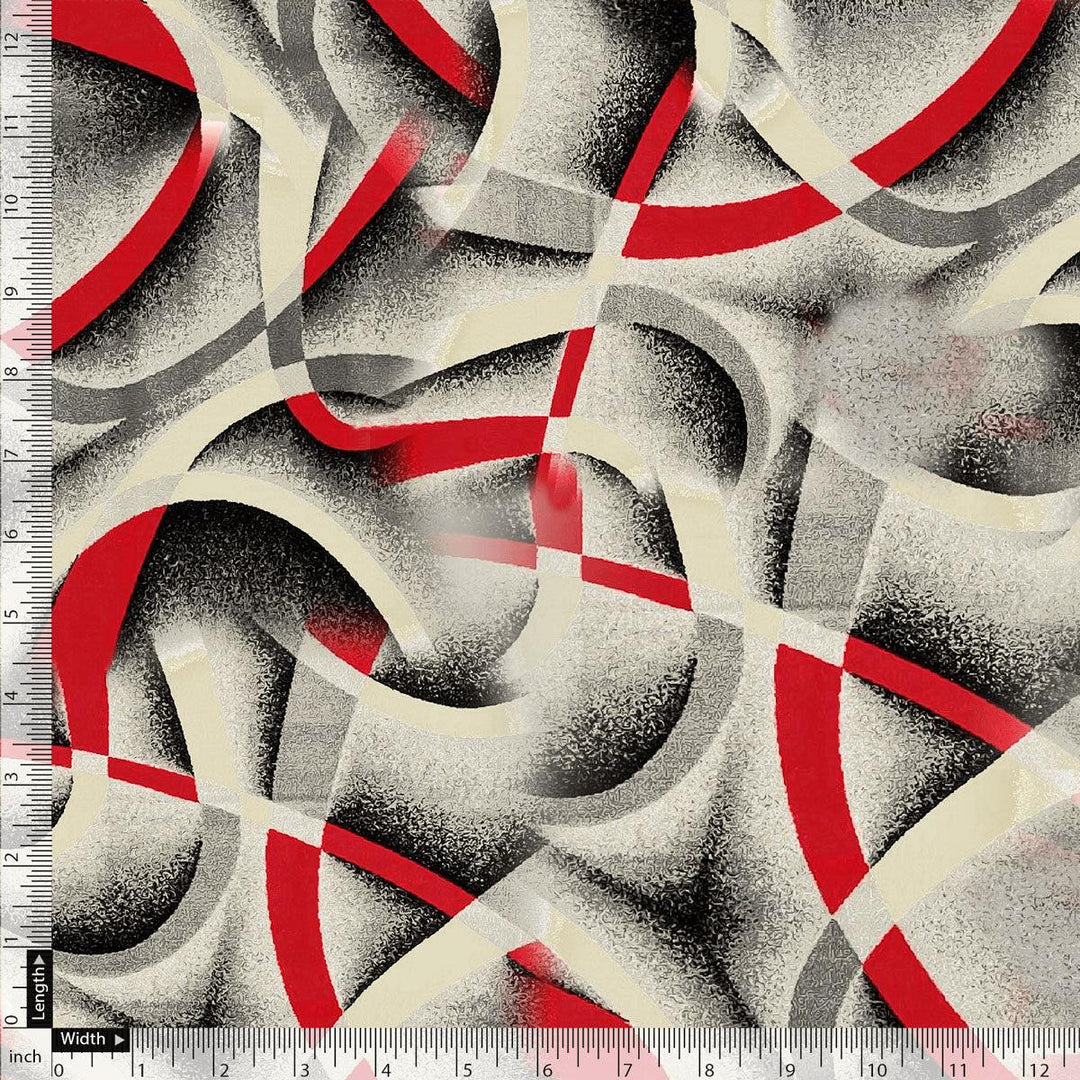This image portrays a square modern art painting characterized by its abstract style. Measuring approximately twelve and three-quarter inches on both sides, indicated by rulers on the left-hand vertical and bottom horizontal edges, the artwork effectively utilizes a mix of colors—predominantly black, gray, white, and red. The composition features amorphous, tunnel-like shapes with red accents outlining their edges, while the interiors transition from black to dark gray, giving them depth and form. The design includes an interplay of color bands that interweave across the canvas, creating a complex network of overlapping and crossing stripes reminiscent of roadways. This pattern is enhanced by a dot technique, providing a textured gradient from densely packed dark areas to lighter, sparser regions, contributing to the overall abstract nature of the piece.